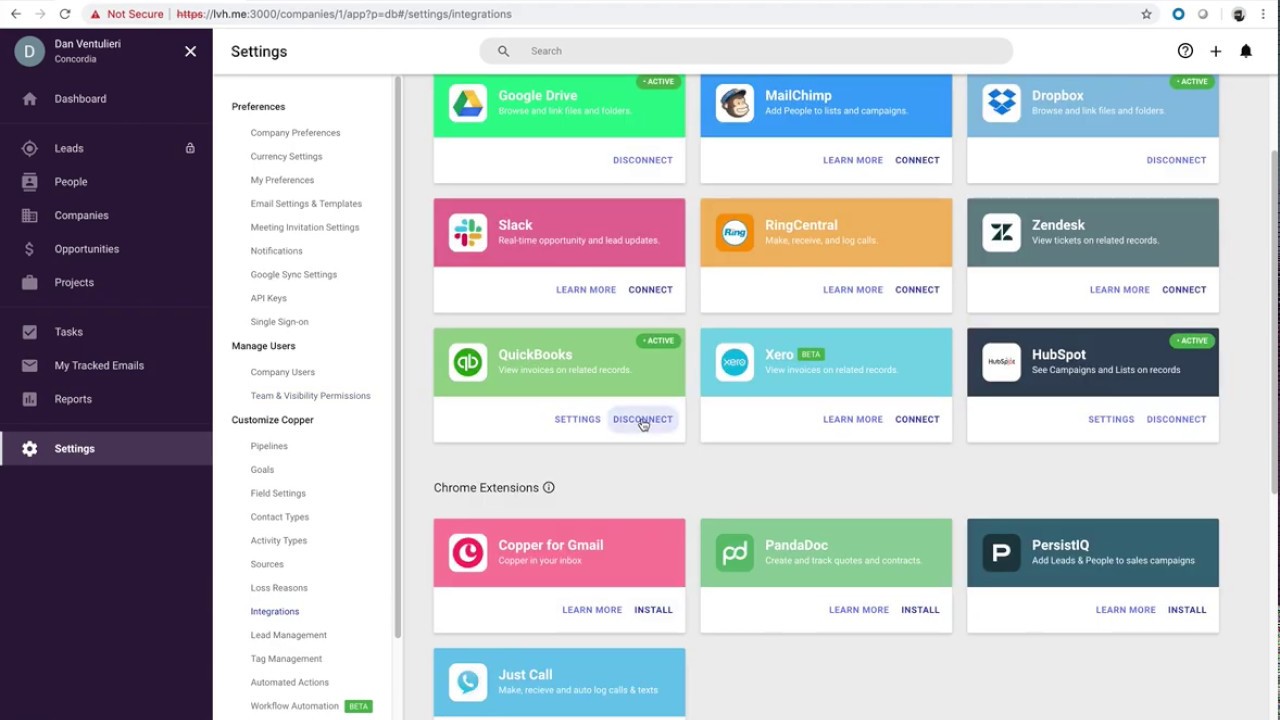This screenshot appears to be from a webpage on the fvh.me website, possibly displaying a user account interface. The layout features a prominent menu bar on the left side with several navigation items: Dashboard, Leads, People, Companies, Opportunities, Projects, Tasks, My Tracked Emails, Reports, and Settings. The 'Settings' item is currently highlighted, indicating that the user is in the settings section.

The main content area showcases a grid of integration options, designed to allow users to connect their accounts with various third-party applications. These options are displayed in multiple rows. The first row includes icons for Google Drive, MailChimp, and Dropbox. The second row features Slack, RingCentral, and Zendesk, followed by QuickBooks and Xero (spelled X-E-R-O) in the subsequent row. Next, HubSpot appears, and a label for Chrome Extensions follows. The grid then lists Copper for Gmail, PandaDoc, PersistIQ, and JustCall as the final integration options.

The organized layout and comprehensive list of apps suggest a robust system for integrating various productivity and communication tools, enhancing the functionality for users managing multiple platforms.